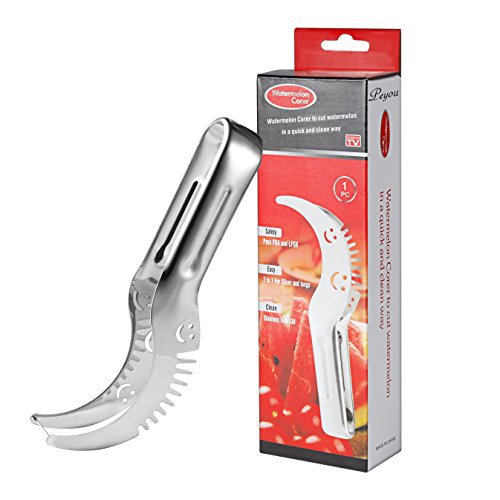The image depicts a specialized tool designed for cutting watermelons efficiently and cleanly. The tool is a unique piece of kitchen equipment, resembling a curved spatula or sickle, crafted from silver metallic material. Its design includes interesting grooves on the back of the blade, and it also functions as a pair of tongs, with the bottom part of the jaws featuring tines and the top part being flat but curved. The accompanying packaging is gray and red with a black stripe along the top, and includes a peg hook slot for store display. The packaging features the brand name "Peyou" and explains that the tool is a watermelon corer. This tool is shown both inside and outside the package, highlighting its dual function and elegant design tailored specifically for cutting and handling watermelon.